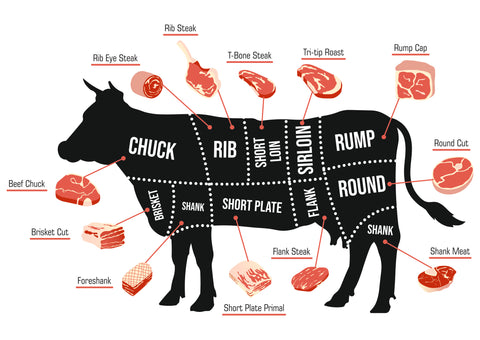This image is a detailed drawing set against a white background, depicting a diagram of the different cuts of meat obtained from a cow. It features a silhouette of a cow with the head and horns facing to the left and the tail to the right. The cow is divided by a series of dotted lines, each section labeled with the corresponding cut of meat and accompanied by small images of the meat for visual reference. 

From left to right, starting at the shoulder, the labeled cuts include the beef chuck, brisket cut (located just beneath the shoulder), and the foreshank (above the front legs). Moving along the body, the cuts include the rib (above the short plate), short plate (near the cow's belly), and flank steak (slightly right of the back legs). Above the flank steak, additional sections such as the short loin, T-bone steak originating from the short loin, and rib eye steak from the rib are identified. Towards the rear end, the rump (connected to the tail) and rump cap (a cut from the rump) are marked, followed by the round section, located just above the back legs, which includes the round cut. The diagram also identifies the rear legs as containing the shank, with shank meat located just above where the two legs form a V. The entire illustration provides a comprehensive view of the cow's anatomy related to its meat cuts, enhancing understanding with marked sections and descriptive labels.